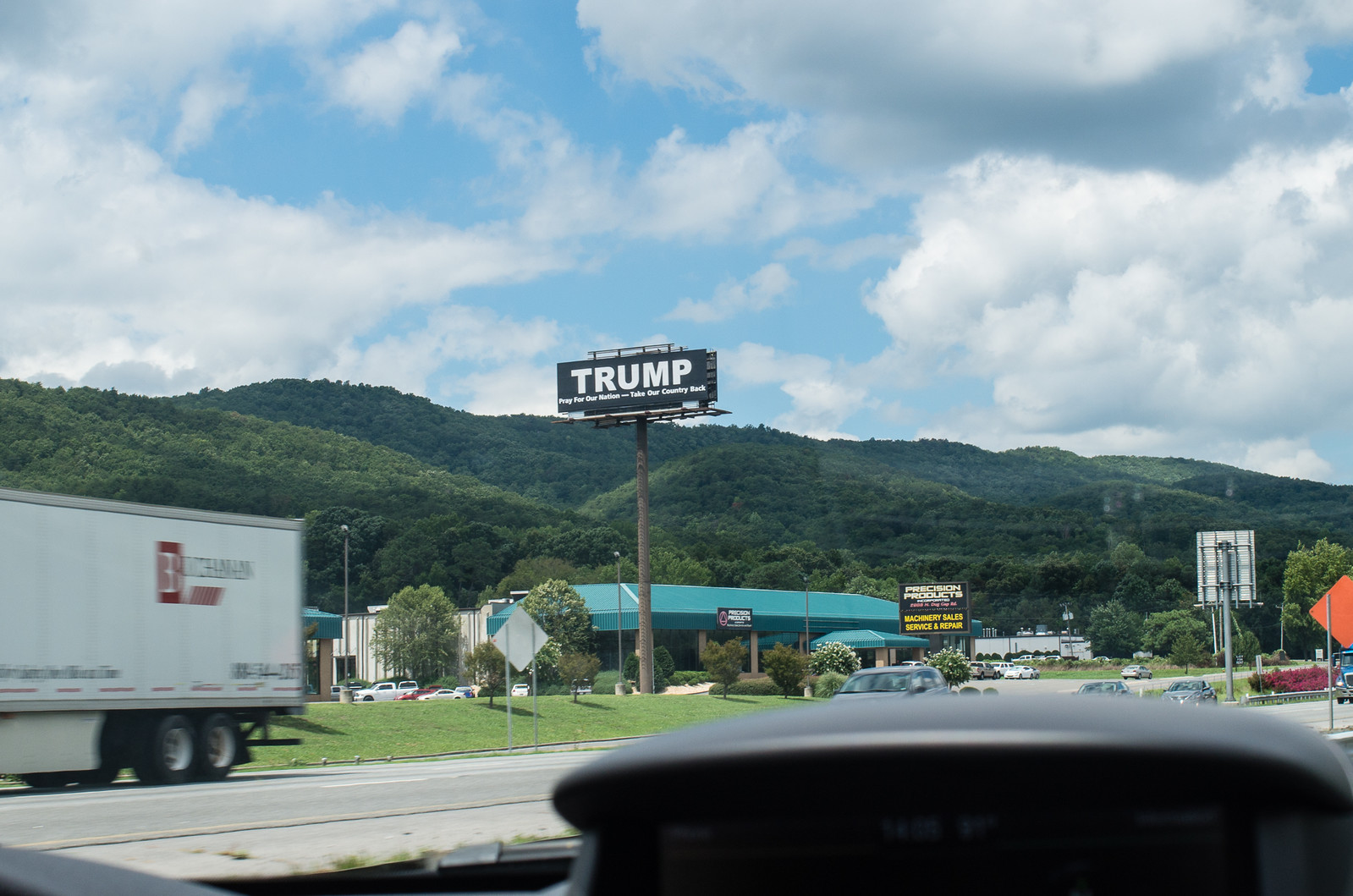This photograph captures a detailed roadside scene taken from the inside of a car, with the dashboard just visible at the bottom of the image. Through the windshield, the scene unfolds under a mostly cloudy blue sky. Rolling green hills covered in forests create a picturesque backdrop. Directly ahead, a two-level building with a turquoise roof sits across a grassy area from the road, which appears to be a truck stop or retail development. The parking lot in front of this building contains various cars, and another building with a similar roof is partially obscured by a large semi-truck. This semi-truck, with a white trailer and black and red logo, is moving towards the camera, along with several other vehicles including another truck with a dark blue cabin. A notable feature is a tall billboard about 50 feet in the air, positioned on a post in the grassy area. The bold black billboard reads "Trump" in white capital letters, with smaller text below that is unreadable from this distance. Additionally, an orange road sign and a barely readable sign, possibly indicating "precision products," add to the mix of visual elements. The photo, taken during the day, combines elements of nature, commercial business, and transportation in a busy, yet scenic roadside vista.